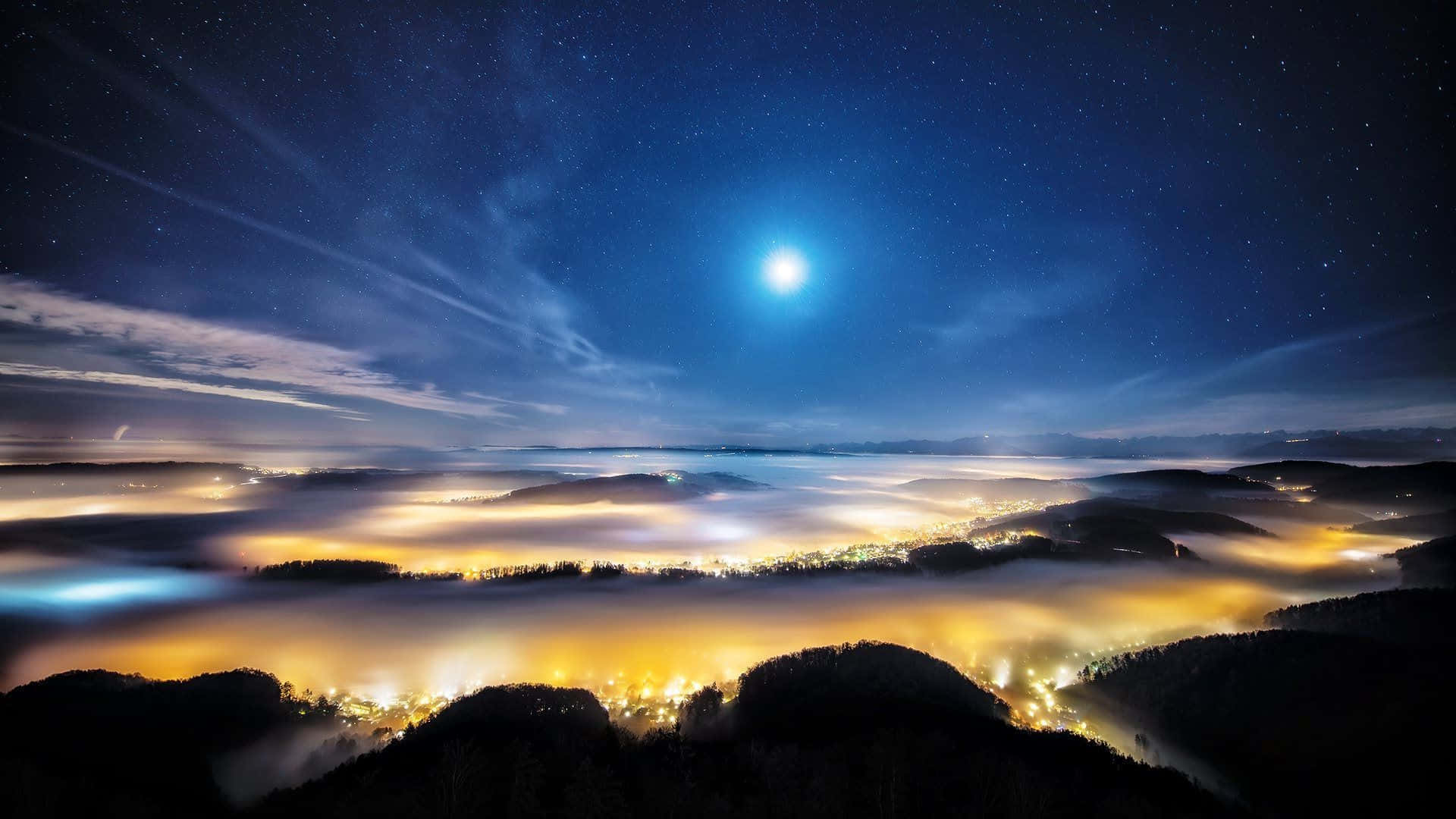An ethereal nighttime photograph captures a serene Swiss landscape under a full moon. The sky transitions from light blue to dark blue with wispy clouds mostly on the left side. A glowing white moon, surrounded by a faint blue halo, occupies the center. The foreground reveals black hills that extend into a misty valley, bathed in a soft yellow glow, likely from city lights below. This mist creates a half-circle arc stretching from the left to the middle right of the image. Within the misty expanse lies a dark, almost circular landmass that resembles an island or the top of a volcano. The scene is further animated by occasional blue hues and scattered stars, enhancing the otherworldly atmosphere. The absence of clear structures due to the enveloping fog adds to the image's dreamlike quality, making the illuminated terrain appear almost celestial.